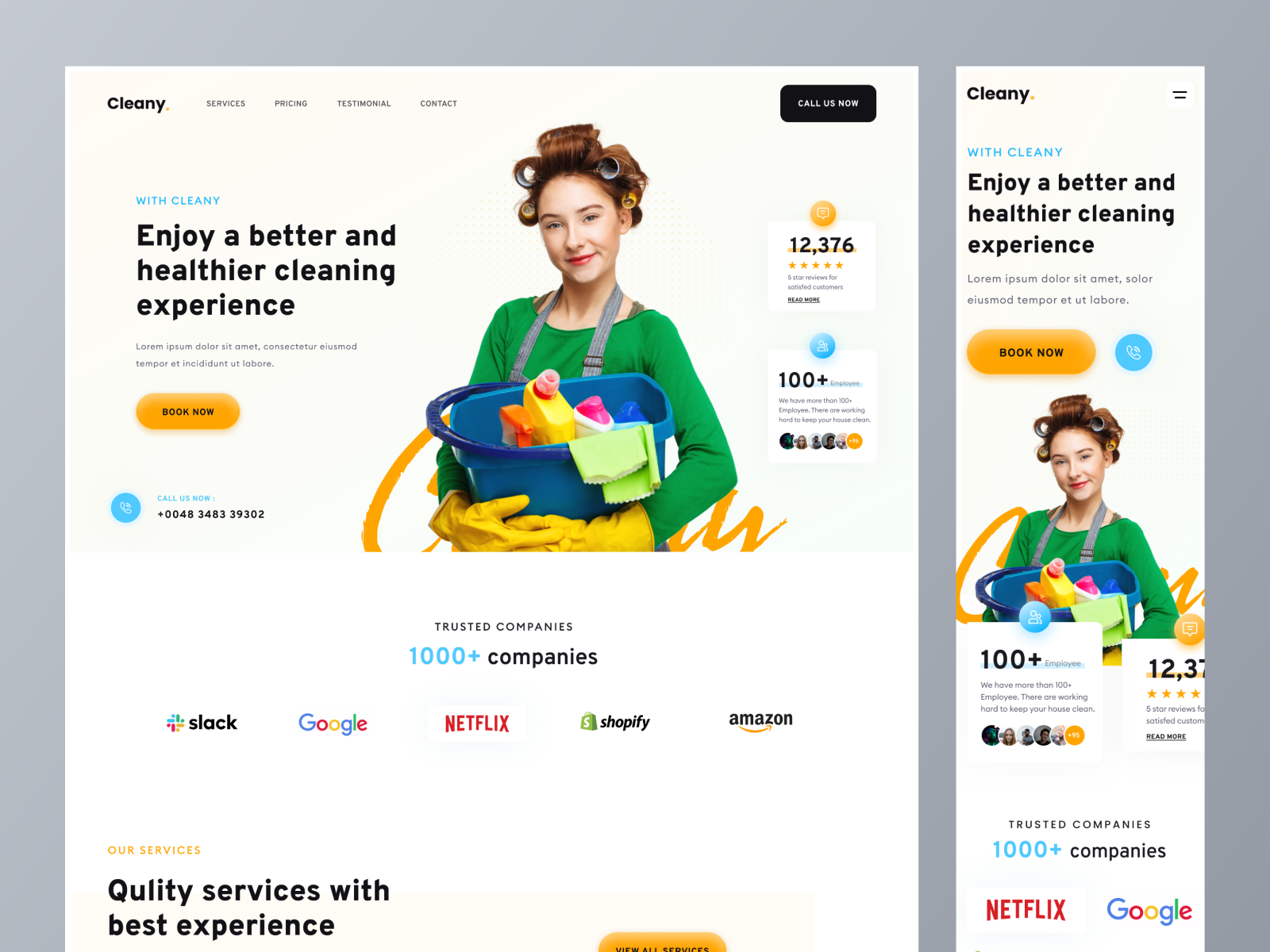Screenshot of Kleeney.com Website

The screenshot depicts the homepage of Kleeney.com. At the top left corner, the logo "Kleeney" is prominently displayed in bold, black lettering. Adjacent to the logo, there are navigation links for "Services," "Pricing," "Testimonials," and "Contact," rendered in a lighter gray font for easy readability.

In the far upper right-hand corner, a black bar featuring the prompt "Call us now" in white lettering is visible. Directly below this bar, the slogan "With Kleeney, enjoy a better and healthier cleaning experience" is presented in eye-catching blue text. An incomplete placeholder text follows, reading: "Lorem ipsum dolor sit amet consectetur adipiscing elit."

Beneath the introductory text, a standout yellow button labeled "Book Now" in black lettering invites users to take action. Nearby, a statistic boasts "12,376 five-star reviews" alongside an assertion that these are "five-star reviews from satisfied customers." Another line mentions that Kleeney employs "100+ employees who are working hard to keep your house clean."

The image also features a photograph of a woman with curling rollers in her hair, wearing a green shirt and overalls. She's holding a blue bucket filled with cleaning supplies and green rags and is equipped with yellow cleaning gloves.

Additionally, the site touts "1,000+ trusted companies" which include major players like Slack, Google, Netflix, Shopify, and Amazon, all highlighting their quality services supported by notable industry names.

Lastly, there is a right-hand side menu that reiterates much of the same information for easy navigation and accessibility.